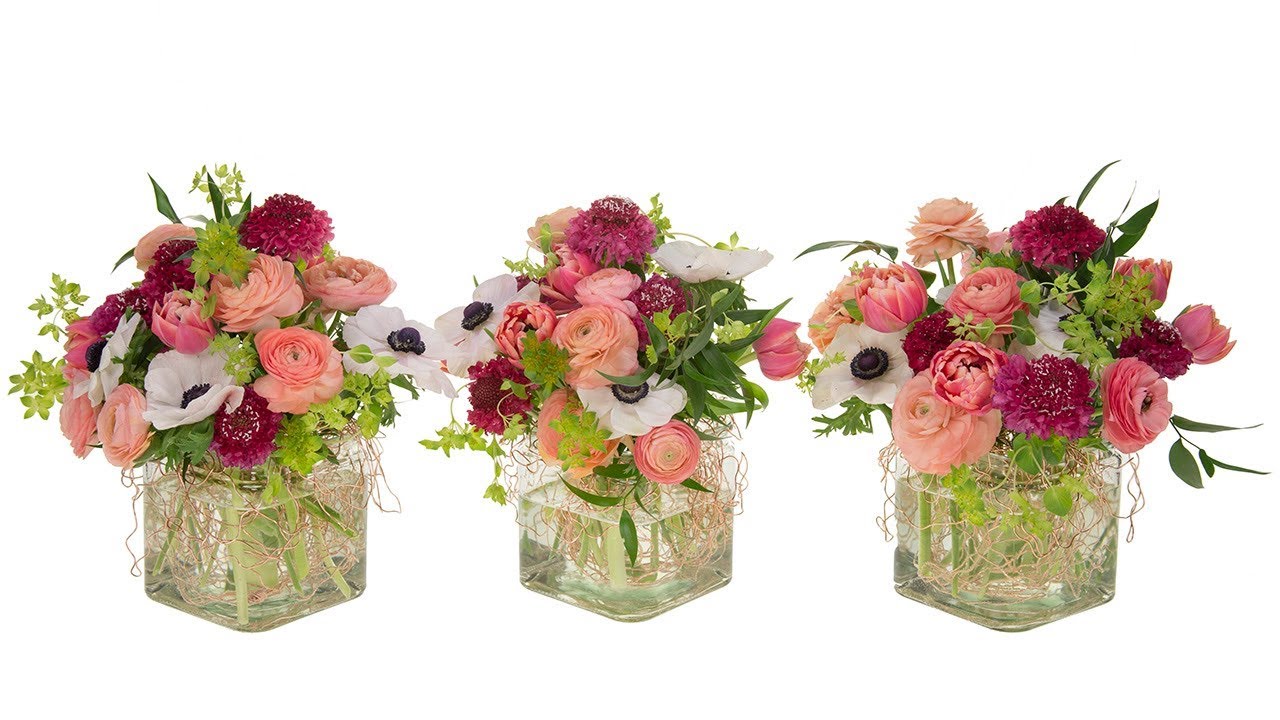The photograph is a horizontally rectangular, full-color image depicting three posed bouquets in transparent square glass vases, against an all-white background. Each vase reveals the green and whitish-colored stems and roots immersed in varying levels of clear water—those on the ends are filled higher than the one in the center. The bouquets are composed of predominantly pink, white, and purple flowers. The white flowers each have a distinctive black circular center. Complementing the main flowers are some that are half-bloomed in pink shades, fully-bloomed lighter pink roses, and purple flowers, some tipped with white. Interspersed throughout the arrangements are sprigs of leafy greenery, with a mix of yellowish-green and darker green leaves that extend from the vases and weave amongst the blooms, giving the bouquets a lush appearance. Despite the slight variations, each bouquet closely resembles the others.